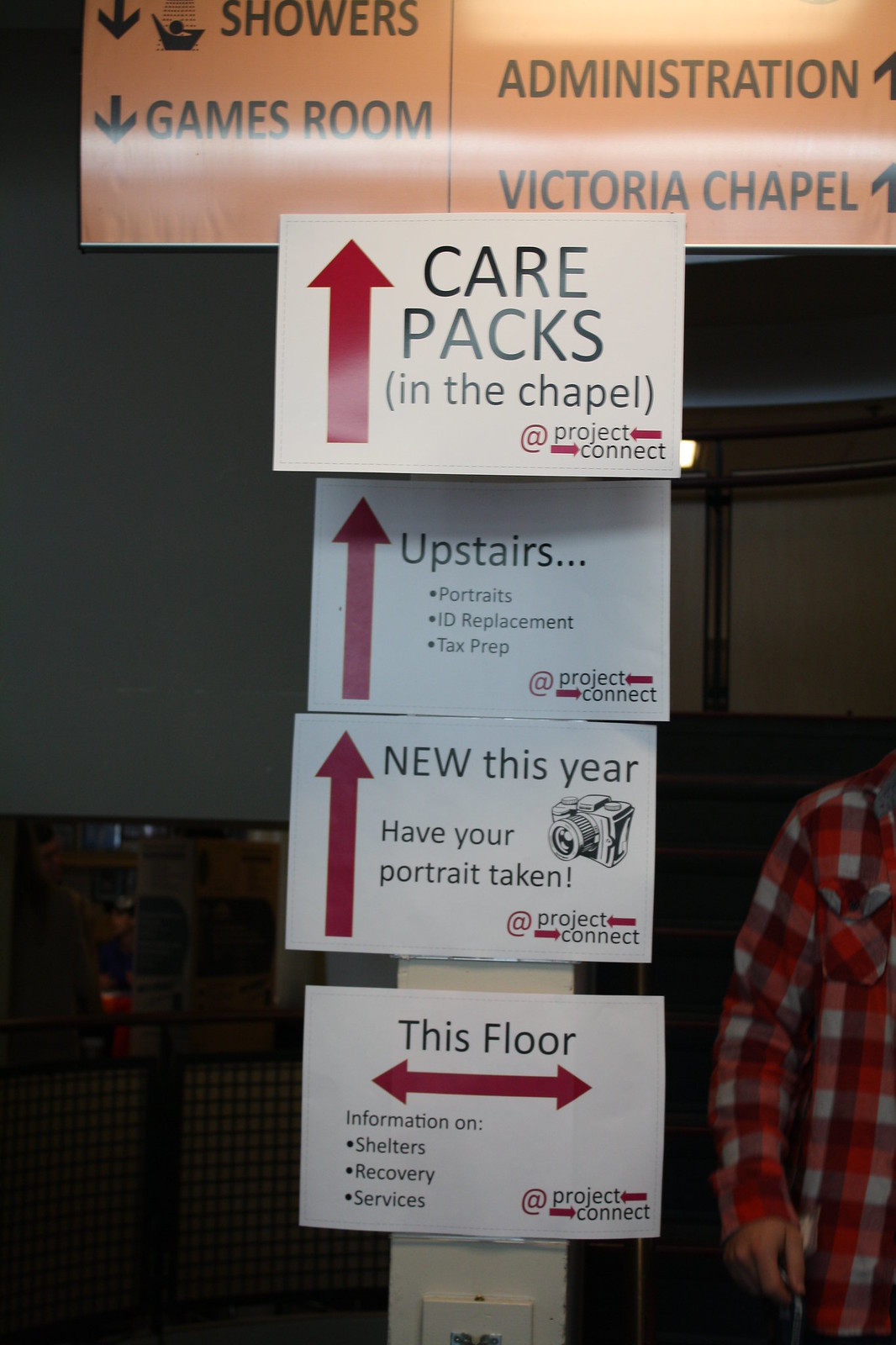A detailed photograph captures a vertical series of signs mounted along the edge of a wall or pillar. At the base, a sign displays the text "This Floor" with a red arrow pointing left and right, indicating "Information on shelters, recovery, and services." Just above, another sign announces "New This Year: Have Your Portrait Taken," accompanied by an image of a camera and a red arrow pointing upwards. Further up, a sign directs attention to services available "Upstairs," including "Portraits, ID replacement, tax prep," with an accompanying upward-pointing red arrow. At the very top, the highest sign reads "Care Packs in the Chapel" also with a red arrow indicating upwards.